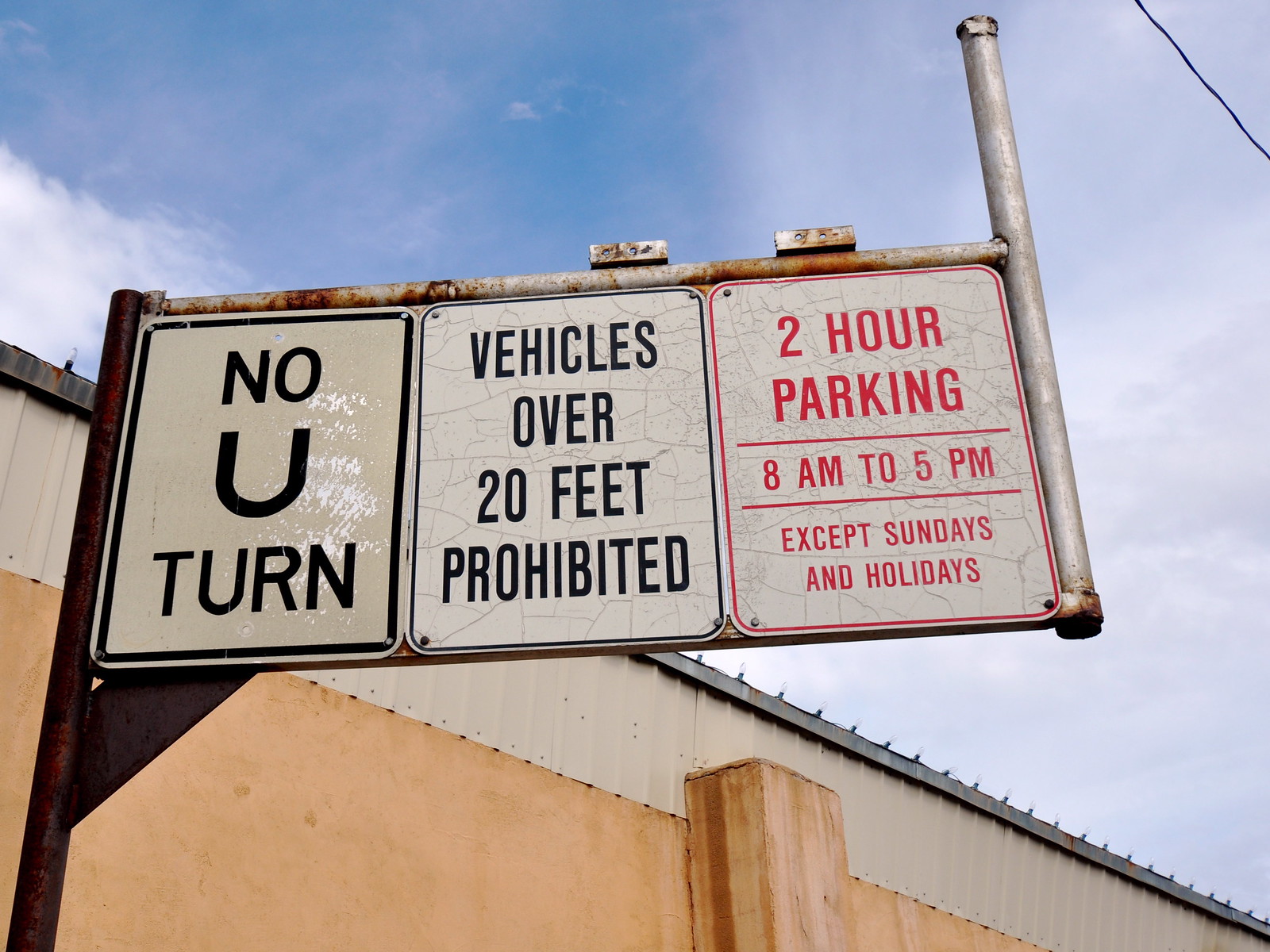The rectangular photograph captures a trio of street signs on an old, rusted metal post against a backdrop of a building and clear blue sky dotted with fluffy white clouds. The focal point, the street signs, are aligned vertically on the post. The top sign, a white one with black trim and black lettering, reads "No U-Turn." Below it, another white sign with black trim states, "Vehicles Over 20 Feet Prohibited." The bottom sign is distinctly different with red trim and red lettering, indicating "2-Hour Parking 8 AM to 5 PM, Except Sundays and Holidays." In the background, a building with a beige stone facade and a tin roof with white and silver sheet metal trim is visible. A power line diagonally crosses the upper right corner, and to the side, a metal pole extends upwards, mounted in the ground. The overall scene is bathed in natural light, enhancing the contrast between the signs and their surroundings.